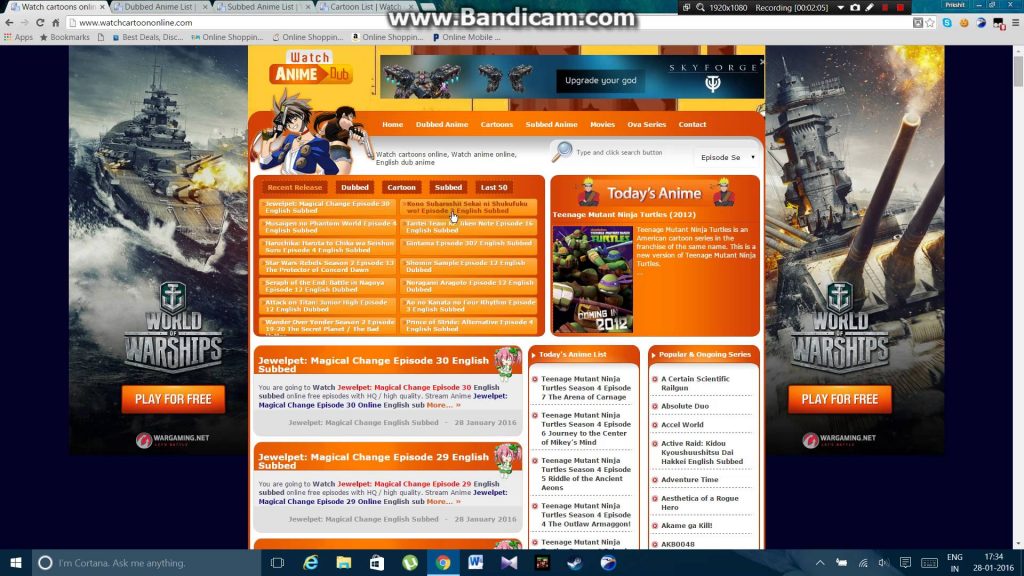The bottom-left section of the image displays a Microsoft Windows interface featuring various icons including Cortana, Internet Explorer labeled with an "e", a shopping bag icon, a "u" symbol possibly indicating uTorrent, Google Chrome, and a "w" symbol among other icons. Additionally, the Steam application is visible. The timestamp reads "17:34:28 21/2016".

The top-left portion of the image has a gray background, while the top section is predominantly black with text indicating "1920x1080" resolution and that it is recording. Below the address bar, the URL www.watchcartoononline.com is displayed.

Various icons and app bookmarks are arranged, showcasing options such as "Best Deals", "Shopping on my Mobile", and "World of War Shows - Play for Free". There's a notable mention of an orange button to "Play for Free".

Further details include text navigation options like "Watch Anyway Dub", "Upgrade Guide", "Home", "Dub to Anime", "Cartoons", "Movies", and "Series". Content highlighted on the page specifies "Today's Anime" with episodes from "Teenage Mutant Ninja Turtles"—specifically Season 4, Episode 2, and Episode 6.